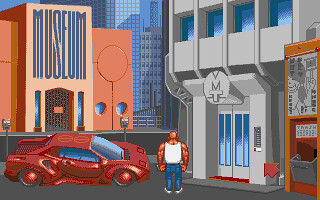The image appears to be a screenshot from an 8-bit style video game, portraying a vibrant, stylized city scene with a clean yet pixelated aesthetic. Dominating the foreground is a muscular, bald man clad in a white tank top, blue jeans, and white shoes, standing centrally between a bright red sports car and a tall gray building adorned with square blue windows and a red-carpeted entrance. The street he stands on is gray, lined with matching gray parking meters. Towering in the far background are gray skyscrapers with numerous white and blue window panels, providing a sense of depth to the urban landscape. Notably, to the left stands a large, terracotta-colored, boxy building marked as a "Museum" in bold gray letters with distinctive circular windows and an arched doorway. On the right, a gold-colored receptacle with a light and dark gray panel and a chute-style door stands prominently, labeled with the word "trash." The scene also includes a red arrow pointing at a door with blue pixel windows and an Eastern text label. The entire frame boasts a blend of modern and retro elements, creating a detailed and immersive snapshot of a digital cityscape.